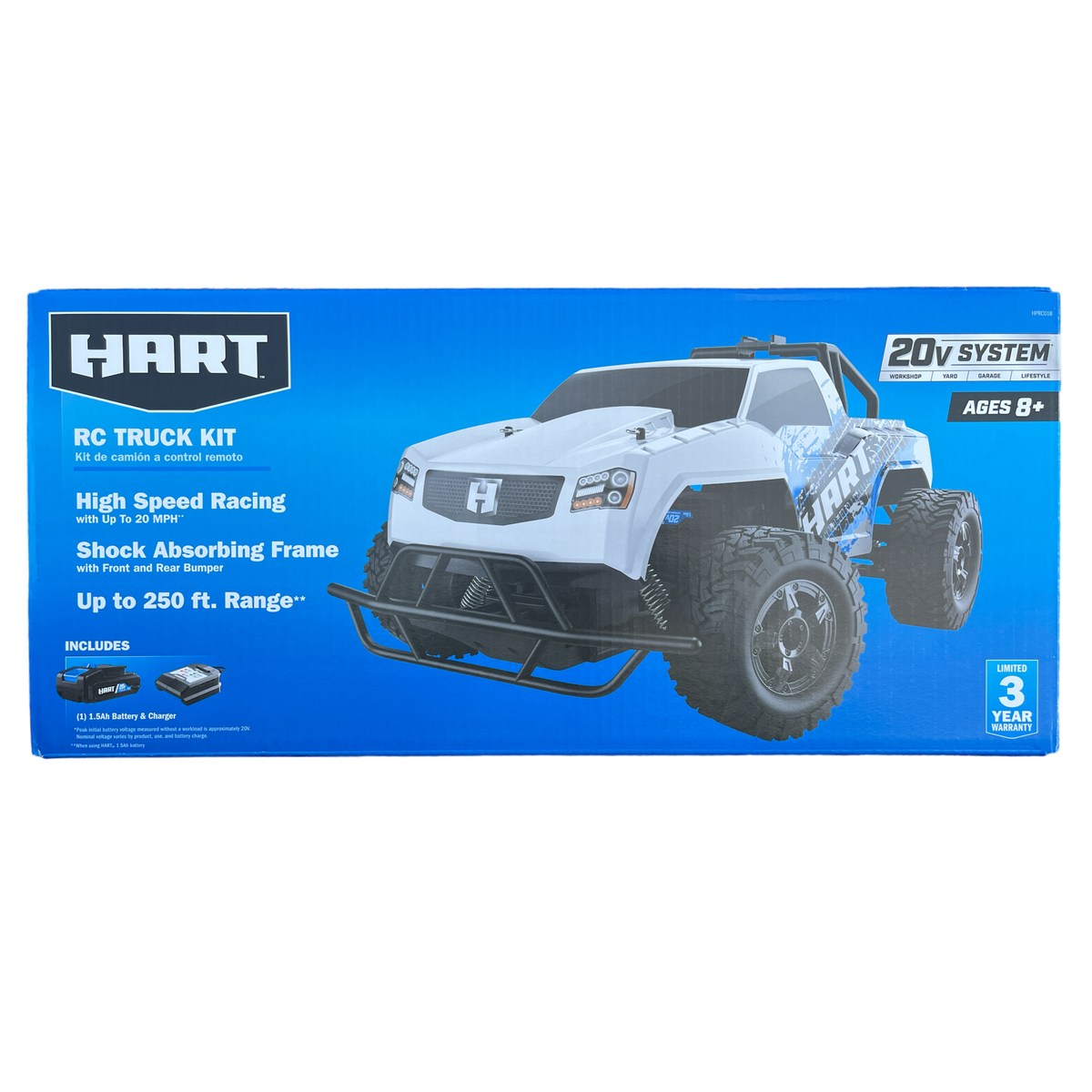The image is of a deep blue cardboard box that prominently features the HART RC Truck Kit on the front. On the left side of the box, the text reads: "HART RC Truck Kit" followed by "High-Speed Racing, Shock-Absorbing Frame, up to 250 feet range. Includes battery and charger." The right side showcases a large, white remote control toy truck with black accents, four large black race tires, and a big metal bar at the back. Details, such as a letter "H" on the front of the truck and pipes below the front grille, add to its robust appearance. Additional information on the top right corner of the box states, "20 volt system, ages 8+, limited 3-year warranty." The overall design signifies a high-performance racing toy suitable for children and hobbyists alike.